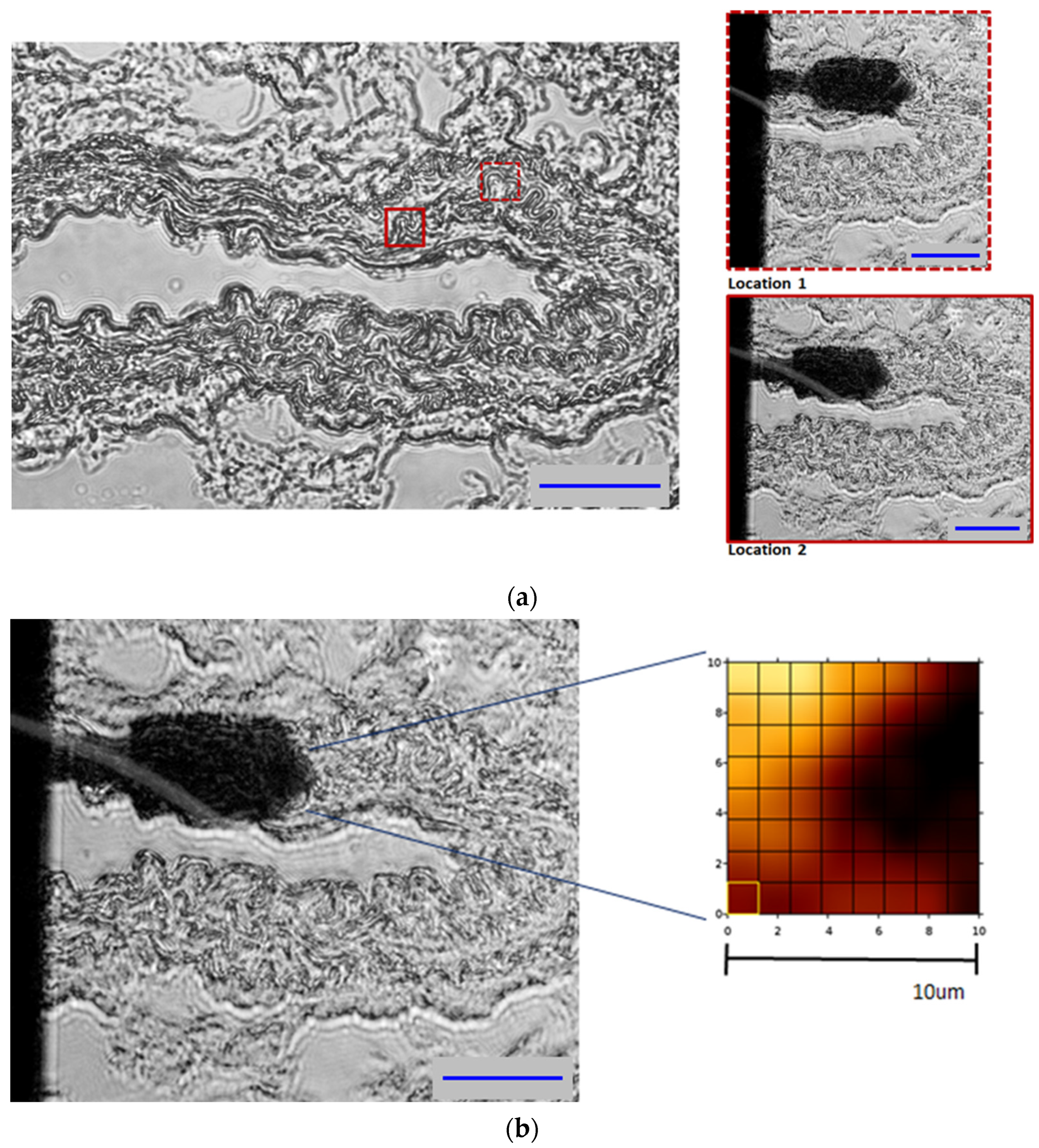The image is a detailed scientific diagram presented on a solid white background. It features multiple frames that collectively illustrate cells under a microscope, primarily in grayscale with some red accents. 

On the top left is a large square frame displaying a complex pattern resembling oil on water with swirled, film-like textures, and it includes two red squares. Adjacent to this, on the top right, are two smaller frames: one zooms in on a shadowed portion of the pattern labeled "location one" within a dashed red border, and another extends this area in more detail labeled "location two," with a solid red border.

Below, on the bottom left, there's another large square that mirrors the top left image but with added emphasis on the shadowed areas. The bottom right contains a smaller, detailed view of the shadow, akin to a microscopic close-up. Next to it, on the far right, is an educational illustration of a heat map, transitioning from yellow to dark brown, displaying a color scale with intensity levels from 1 to 10 to represent heat variations.